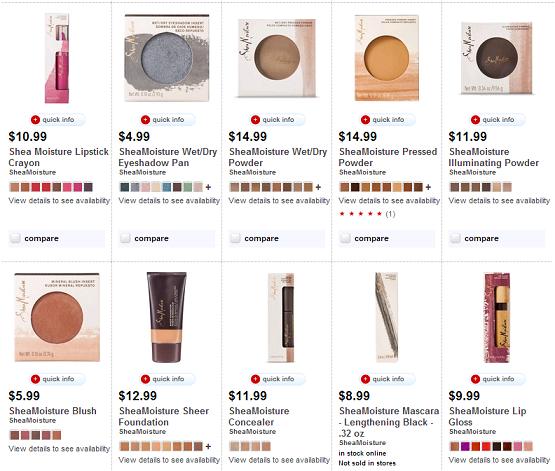On a sleek white background, the webpage showcases a neat and visually appealing layout perfect for browsing makeup products. A delicate gray line graces the top of the page, providing a modern touch. Below this line, the products are displayed in a well-organized grid spanning across two rows, each consisting of five images. Thin gray lines vertically and horizontally separate the images, ensuring a clean and structured presentation.

Each product image is meticulously detailed. For instance, the first product features a gradient pink box with the lighter shade on the top maturing into a darker hue towards the bottom, containing an exquisite lipstick. Directly below each image, a small white tab on the left side sports a red circle with a white plus sign, marked with the text "Quick Info" in black. 

Proceeding downward, the price of the product is indicated, followed by the product name and the manufacturer's details. Eight small color swatches beneath each product display the variety of available shades. Below these swatches, the phrase "View Details to See Availability" is printed in black, inviting further exploration.

A subtle grey tab at the bottom features a white circle with the word "Compare" in black, allowing users to compare different products. Notably, the fourth item in the bottom row stands out with the unique label "In Stock Online, Not Sold in Stores" in lieu of the usual availability details.

Overall, this clean and detailed layout ensures a seamless and informative shopping experience for makeup enthusiasts.